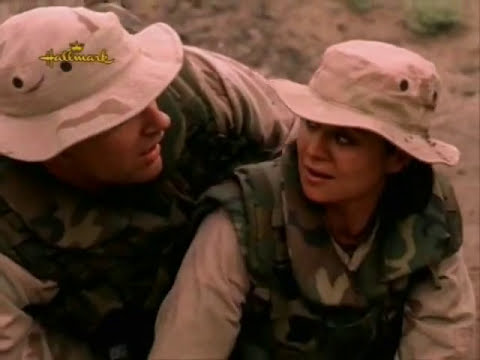The image is a screenshot from a Hallmark movie, as indicated by the Hallmark logo, which appears in the upper left corner in gold script with a crown. It features a close-up of a man and a woman dressed in matching military attire. Both are wearing khaki-colored army fatigues, long-sleeved shirts, and camouflage vests in green and brown tones. They also sport khaki-colored fishing hats with short brims. The man, positioned slightly behind the woman and to the left, has his arm extended behind her as they both kneel on the ground and gaze at each other. The background shows a rocky, sandy area with sparse vegetation, including patches of green grass and plants.